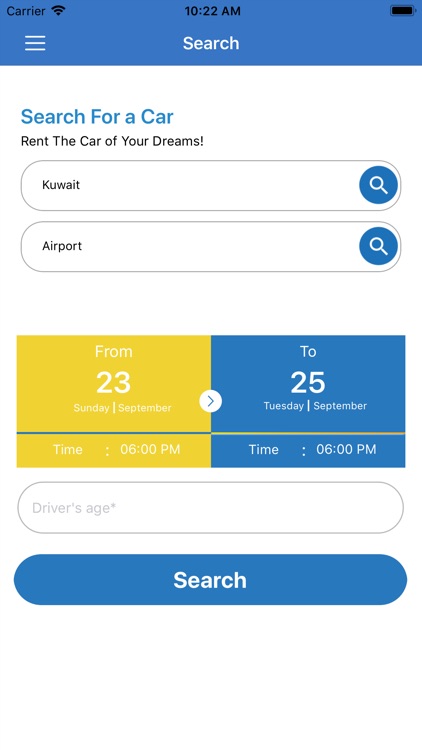The image displays a computer screen with a user interface designed for renting cars. At the top, within a blue header bar, there is a label that reads "Just Carrier," though it doesn't mention a specific name. The time is shown as 10:22 a.m., and the battery is fully charged. The blue bar also includes a search bar and a menu icon comprised of three horizontal lines.

Below the blue header, the interface has a white background. At the top, it prominently states in black text: "Search for a car. Rent the car of your dreams!" followed by an exclamation point.

In the example provided, "Kuwait" is entered in the search bar, with an option to specify a pickup and drop-off location, such as an airport. A yellow box labeled "From" indicates the rental period, showing dates from Sunday, September 23rd to Tuesday, September 25th, with both pickup and drop-off times set at 6:00 p.m.

Below this, there is a white box outlined in gray asking for the driver's age, marked with an asterisk indicating that it is a required field. At the bottom of the interface is an oval blue "Search" button that users can click to find available cars and prices, enabling them to rent the car of their dreams.